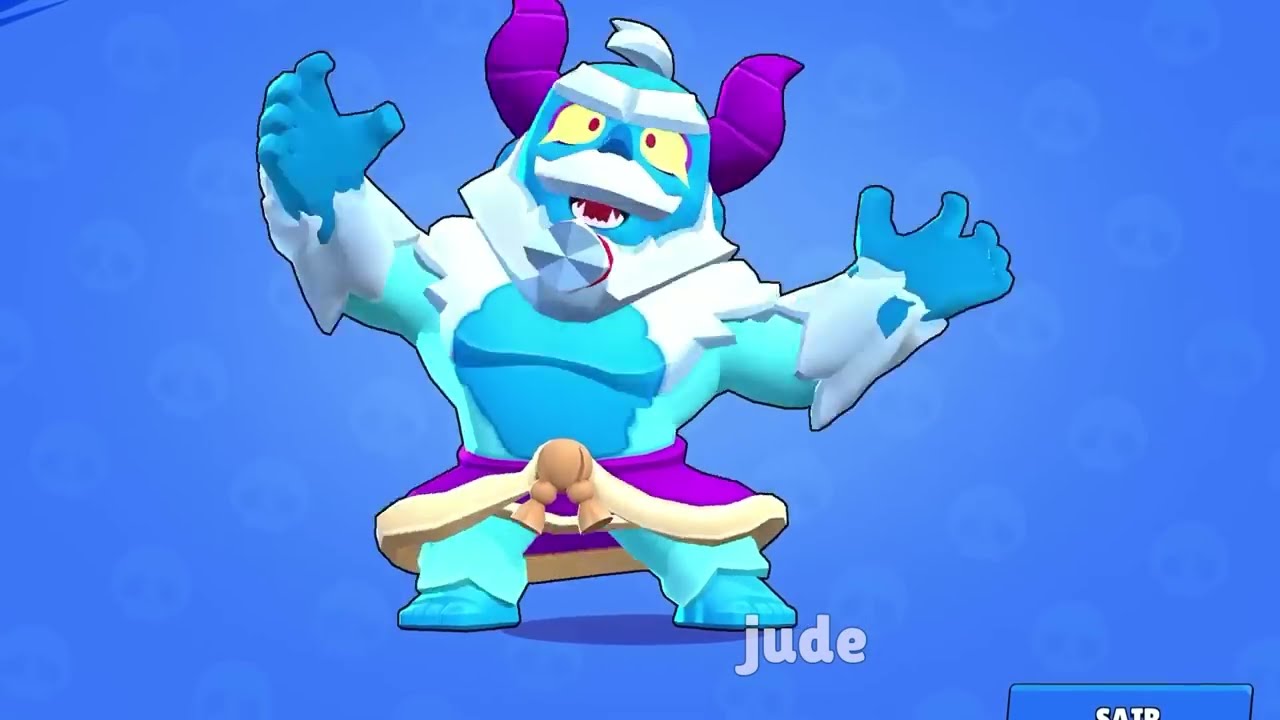The image features a cartoon character named Jude, a quirky and somewhat menacing snowman-like figure with an abominable snowman or yeti appearance. Jude stands against a light blue background adorned with faint circles, resembling ghostly heads. He has distinct purple horns with two horizontal lines each, jutting out from his head. His face is white, with striking yellow eyes and red pupils, framed by square white eyebrows. Beneath the eyebrows, he sports a square white mustache with a flat bottom. His mouth is open wide, revealing sharp teeth and a red interior.

Jude's upper chest displays a mixture of light and dark blue colors, while his shoulders are adorned with fur-like white segments resembling ice. His outstretched arms, with the left arm slightly higher, end in blue hands surrounded by icy white wristbands. Around his waist, Jude wears a purple skirt-like garment with a yellow lining at the bottom, along with blue pants and darker blue boots.

Underneath Jude's right foot is the name "Jude" inscribed in all lowercase letters. In the bottom right corner of the image, there's a partially visible blue square containing the letters "S-A-T-R," which are cut off at the bottom. Jude's robust and short stature, coupled with his eerie grin, sharp teeth, and unusual attire, make him the focal point of this peculiar and vividly detailed cartoon depiction.